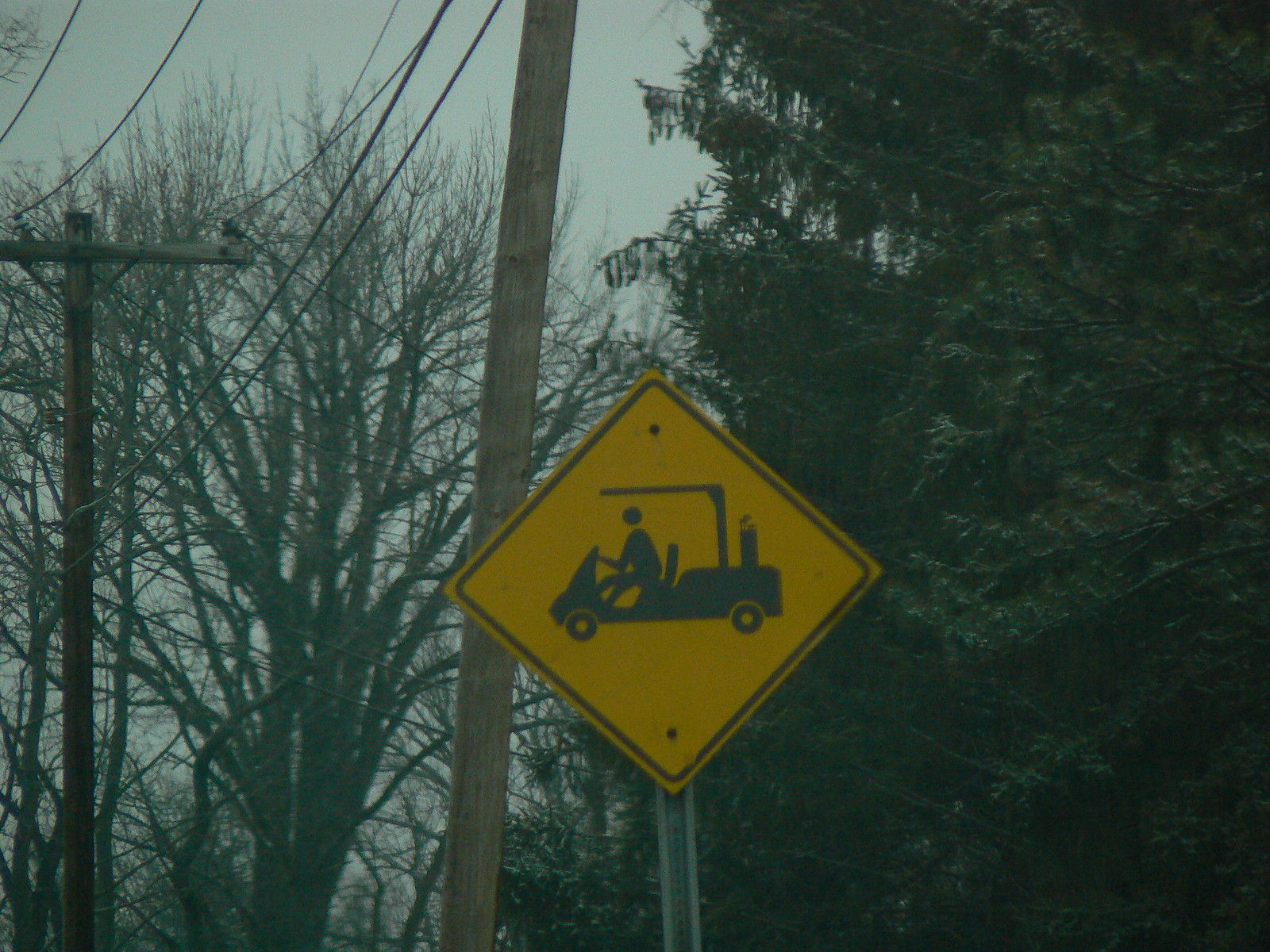The close-up image captures a triangular yellow street sign depicting a silhouette of a person seated in a golf cart, with an object in the back, indicating a designated golf cart crossing area. Dominating the right half of the picture is a lush, dark green tree, fully in bloom with thick branches. In contrast, the left half of the image features a gray, winter-like sky and a bare tree devoid of leaves. Additionally, a few utility poles, likely for telephone or electricity lines, can be observed on the left side.